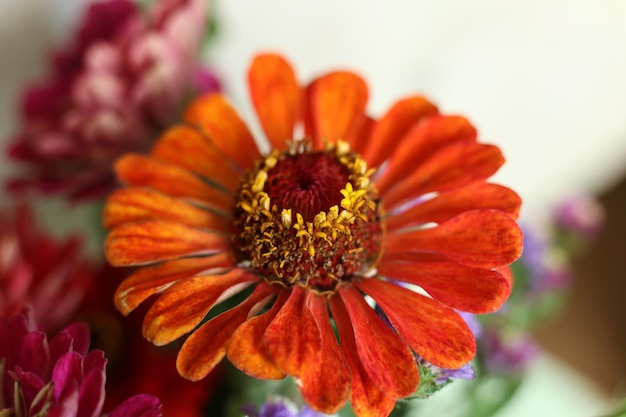This is a detailed macro photograph of a vibrant orange flower, which is the main focus and positioned prominently in the center of the image. The petals are a striking coral color, exhibiting a gradient that transitions to yellow towards the tips. The flower's center is a deep burgundy shade surrounded by a fringed ring of light yellow petals and, at the very core, a bud that combines hues of yellow and maroon. Behind the primary flower, the background is blurred but reveals a variety of other flowers in softer, more muted tones of purple, pink, and white. Among these, a partially closed flower with white-backed petals is noticeable in the top left, while the bottom left corner hints at another flower, probably of the same species but with a pinkish hue. The green foliage and potential presence of a white, possibly faded out table, combined with pink and purple flowers, frame the scene, enhancing the composition without detracting from the central flower's intricate and vivid details.